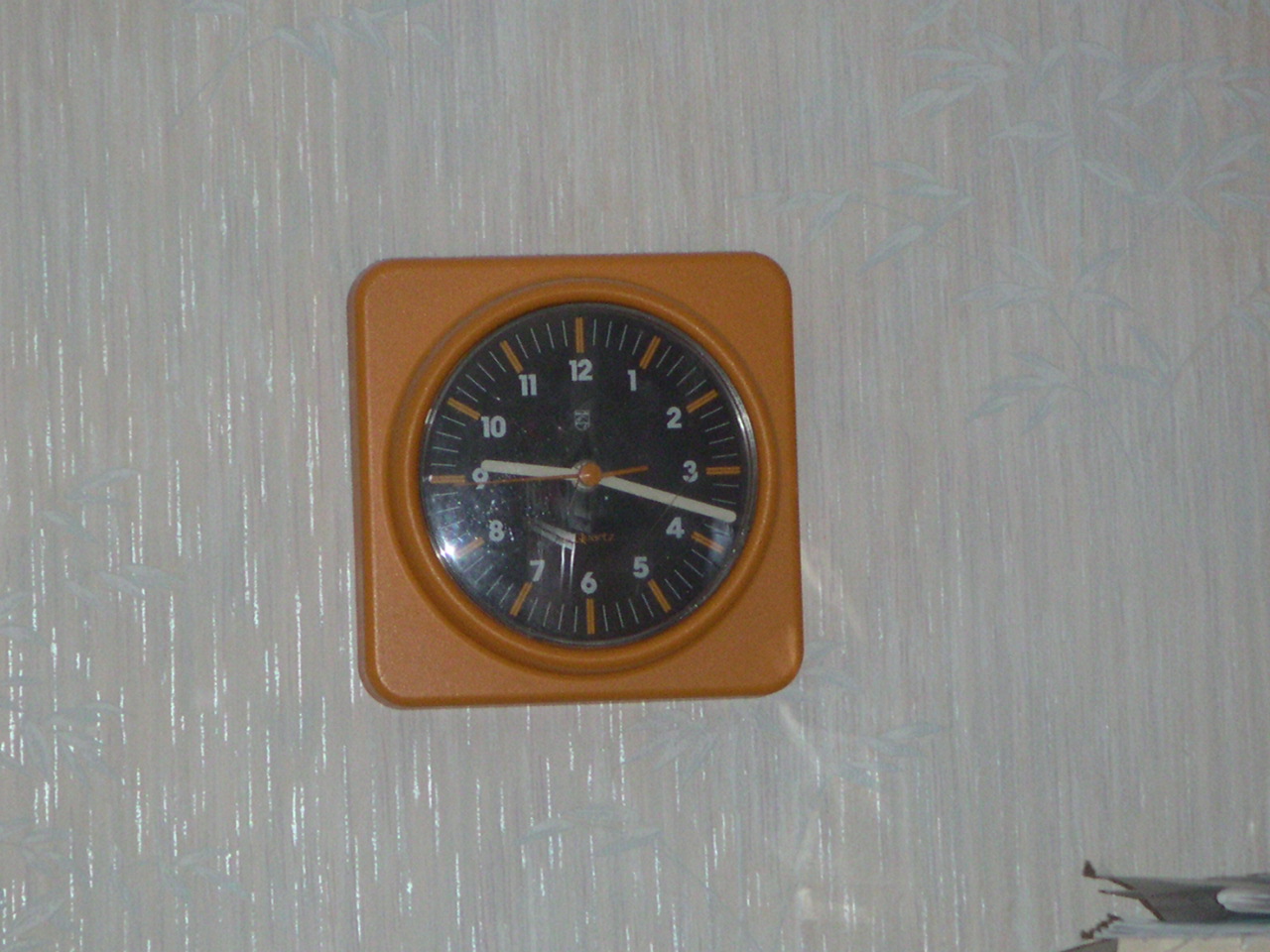The image depicts a vintage-style clock prominently mounted on a white, textured wall with a reflective, shimmery finish. The clock itself is square with rounded edges, crafted from a plastic material in a burnt orange or light brown color. The clock's face is black, and it features white numbers in standard format from 1 to 12, with each hour mark highlighted by an accompanying orange stripe for enhanced readability. The clock has white hour and minute hands and an orange second hand, all pointing to the time of 9:18. In the bottom corner of the image, there is a metallic object extending upward, likely emanating from a table or shelf, slightly visible but difficult to identify.